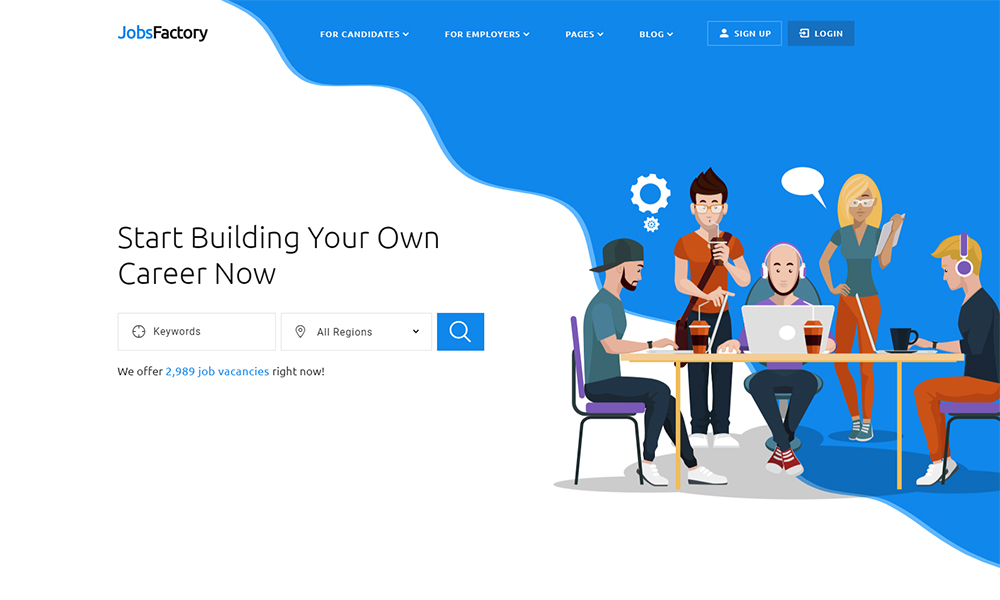This landscape-oriented photo captures a homepage of a website named "Jobs Factory," as indicated by the blue and black logo situated at the upper half of the page. The background is artistically split with a slope-like line, rendering the left side predominantly white and the right side blue.

At the top of the page, a navigation bar features several white drop-down menus labeled "For Candidates," "For Employers," "Pages," and "Blog." Additionally, there are two primary call-to-action buttons on the right side of the navigation bar: a blue "Sign Up" box with white font and a darker blue "Login" box, also with white font.

In the central left section of the page, there's a prominent headline in black font that reads, "Start Building Your Own Career Now." Directly beneath this heading is a search interface, consisting of a text box labeled "Keywords," a drop-down box with a pinpoint icon labeled "All Regions," and a blue search button featuring a yellow or white magnifying glass icon. Just below the search interface, a message informs users, "We offer 2,989 job vacancies right now."

Positioned to the right of this central area is an image featuring five individuals gathered around a table. Three men are seated and working on laptops, while another man stands behind them with a bag over his shoulder. Additionally, a woman is positioned behind the group, next to a thought bubble, adding a dynamic visual element to the scene.